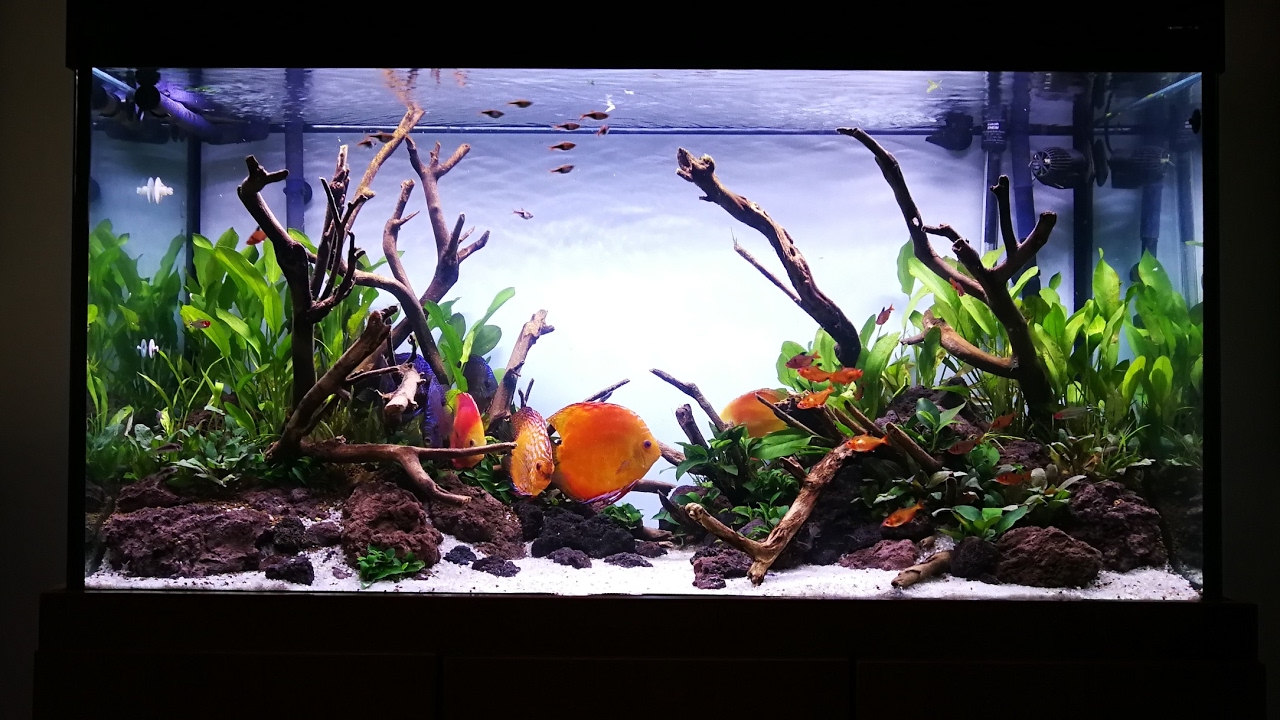This detailed photorealistic image showcases an active and carefully curated aquarium. At the center, a vibrant, large, round orange fish captures the eye, surrounded by a lush underwater landscape of white sand. Intricately arranged branches of driftwood, along with dark brown and gray pieces, are decoratively placed throughout the tank, creating a dynamic, natural environment. Green plants and smaller flora are interspersed in the background and foreground, adding to the aquatic scenery. Scattered brown rocks and lava stone-like items enhance the tank's detailed bottom. Besides the prominent large orange fish, the tank also houses a variety of other fish, including smaller goldfish and a notably colorful fish with pink and yellow hues. A small school of little fish can be seen towards the top, suggesting an active feeding time. The water appears clear, with no visible text in the image, and the close-up focus intensifies the detailed and vibrant underwater scene.